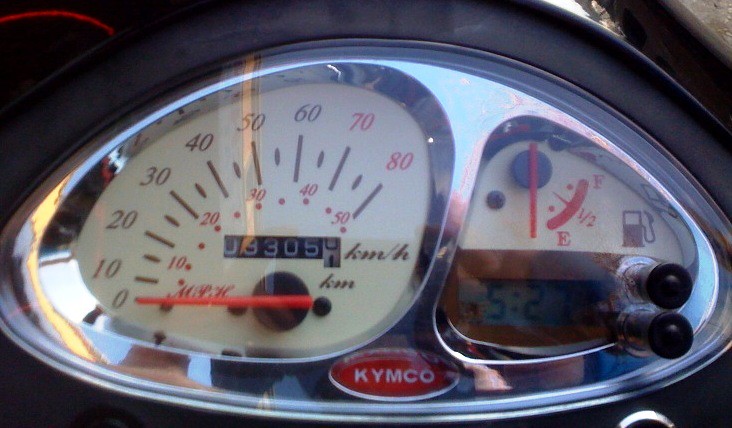This close-up photograph captures the intricate details of an analog instrument panel mounted on a chrome background. Dominating the scene is a large, oval-shaped display with two distinct analog gauges.

On the left side, a gauge features a red needle pointing to a semicircular scale ranging from 0 to 80. The current reading is 0. In the center of this gauge is an inset display showing the numbers "08305."

On the right side, the gauge is topped by a black knob, with a red arrow—likely the indicator—pointing towards a red semicircle at the bottom right position. Above and below this semicircle are the letters "F" and "E," respectively, identifying this gauge as a fuel indicator.

At the very bottom of the instrument panel, the manufacturer's logo, "KYMCO," stands out in white against a red background, adding a distinct brand signature to this sophisticated analog instrumentation.